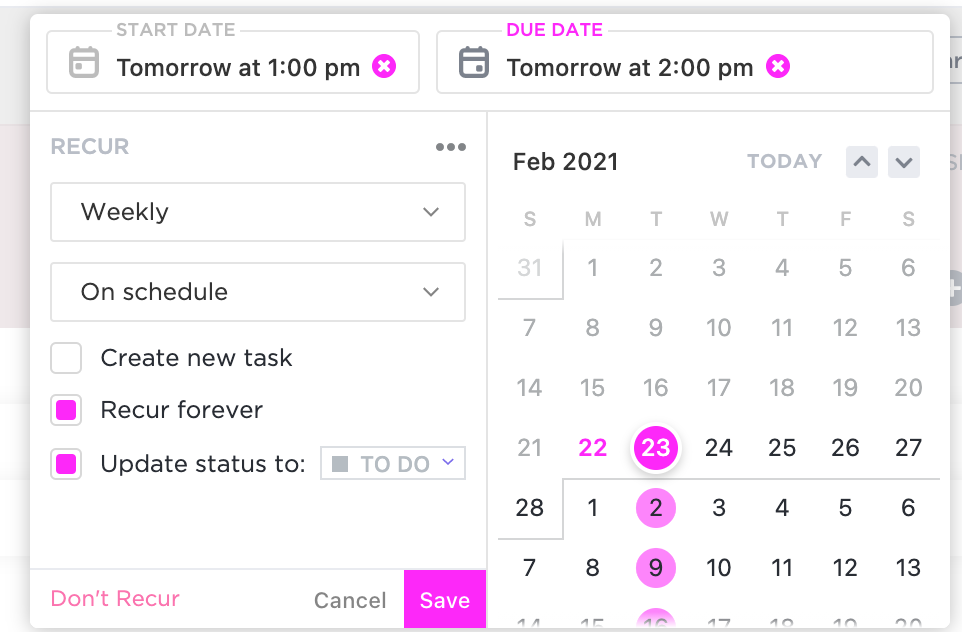The image displays a printout of a task calendar. At the top, it specifies the start date as "Tomorrow at 1 p.m." marked with a purple circle containing a white X. Adjacent to this, in purple lettering, is the label "Due Date," followed below by "Tomorrow at 2 p.m." printed in black with a matching purple circle and white X. 

From left to right on the card, there are several options: "Recur," with a dropdown showing "Weekly," "On Schedule," "Create New Task," "Recur Forever," and "Update Status," the latter two being selected and highlighted by purple squares. At the bottom left corner, "Don't Recur" is displayed in purple. 

To its right, there are options to "Cancel" or "Save," with the word "Save" displayed in white letters within a purple square. The right portion of the image shows a calendar for February 2021 printed in black, starting from January 31st, which falls on a Sunday. The dates 22nd and 23rd of February are highlighted in purple, indicating important or selected dates.